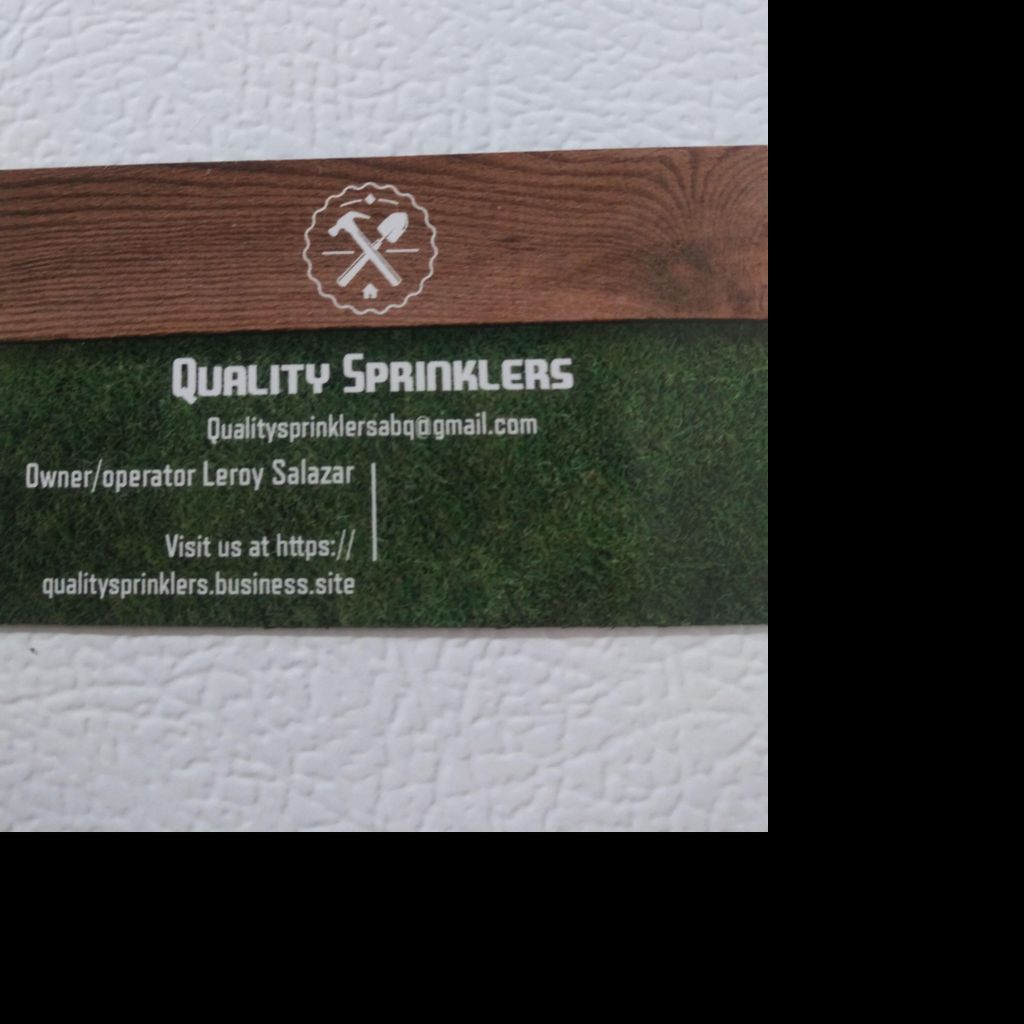The image features an advertisement for a company named Quality Sprinklers. Dominating the upper portion of the image is a white textured wall above a brown, wooden rectangular board, slightly off-center to the top left. The board displays a logo depicting a hammer and a shovel crossed over each other. Below this wooden board, vibrant green grass serves as the backdrop for various text elements. The text includes "Quality Sprinklers" followed by their email, "qualitysprinklersabq@gmail.com," and the name of the owner/operator, "Leroy Salazar." Additionally, there's a call to visit their website at "https://qualitysprinklers.business.site." Framing the left and bottom edges of the image is a large, thick, black area shaped like an inverted L, adding stark contrast to the overall composition. The primary colors present in the ad are white, brown, black, and green, which collectively underscore the advertisement for Quality Sprinklers.